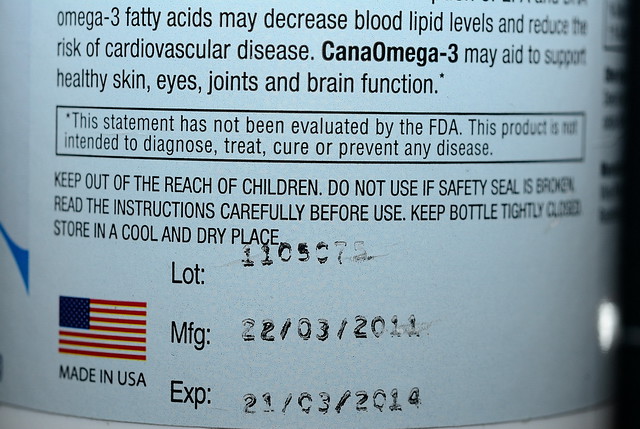This image is an up-close photo of the back label of a white bottle or pot, likely a supplement canister for Canna Omega-3. The label details the product's benefits and safety information. At the top, it describes Omega-3 fatty acids, stating they may decrease blood lipid levels and reduce the risk of cardiovascular disease, as well as support healthy eyes, skin, joints, and brain function. It also contains a disclaimer that says: "This statement has not been evaluated by the FDA. This product is not intended to diagnose, treat, cure, or prevent any disease."

Further down, there are important safety warnings which include: "Keep out of the reach of children," "Do not use if the safety seal is broken," and "Read the instructions carefully before use." Additional storage instructions advise keeping the bottle tightly closed and storing it in a cool, dry place. The bottom part of the label displays manufacturing details, including a lot number (Lot: 1105075), manufacturing date (MFG: 22/03/2011), and expiration date (EXP: 21/03/2014). On the bottom left, there is an American flag graphic with "Made in the USA" written below it. On the right, a thin black border frames the label.